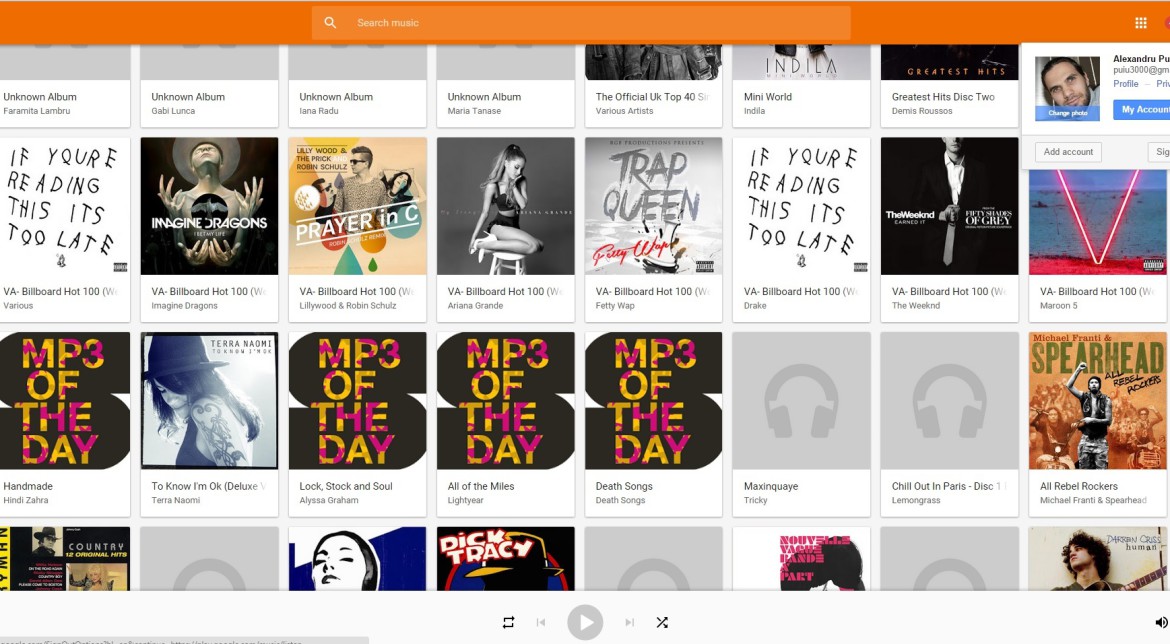The image depicts a web page from a music platform. The top border of the page is highlighted in orange, featuring a search box for music. On the far right, there is an icon consisting of a square divided into nine smaller squares. Below this, there is a list of albums displayed in four rows, each containing eight albums.

Some of the albums are named, while others are labeled as unknown. Among the visible album names are "Imagine Dragons," "Trap Queen," "Sugar," "Spearhead," "MB3 of the Day," "Terra Naomi," "Ariana Grande," and "Dick Tracy." Some album titles are cut off and not fully visible.

The bottom border of the page is light gray and includes a set of media control buttons: a refresh button, a rewind button, a play button, a fast forward button, and another icon that appears to represent tools. Additionally, there is a sound icon indicating that the sound is currently on.